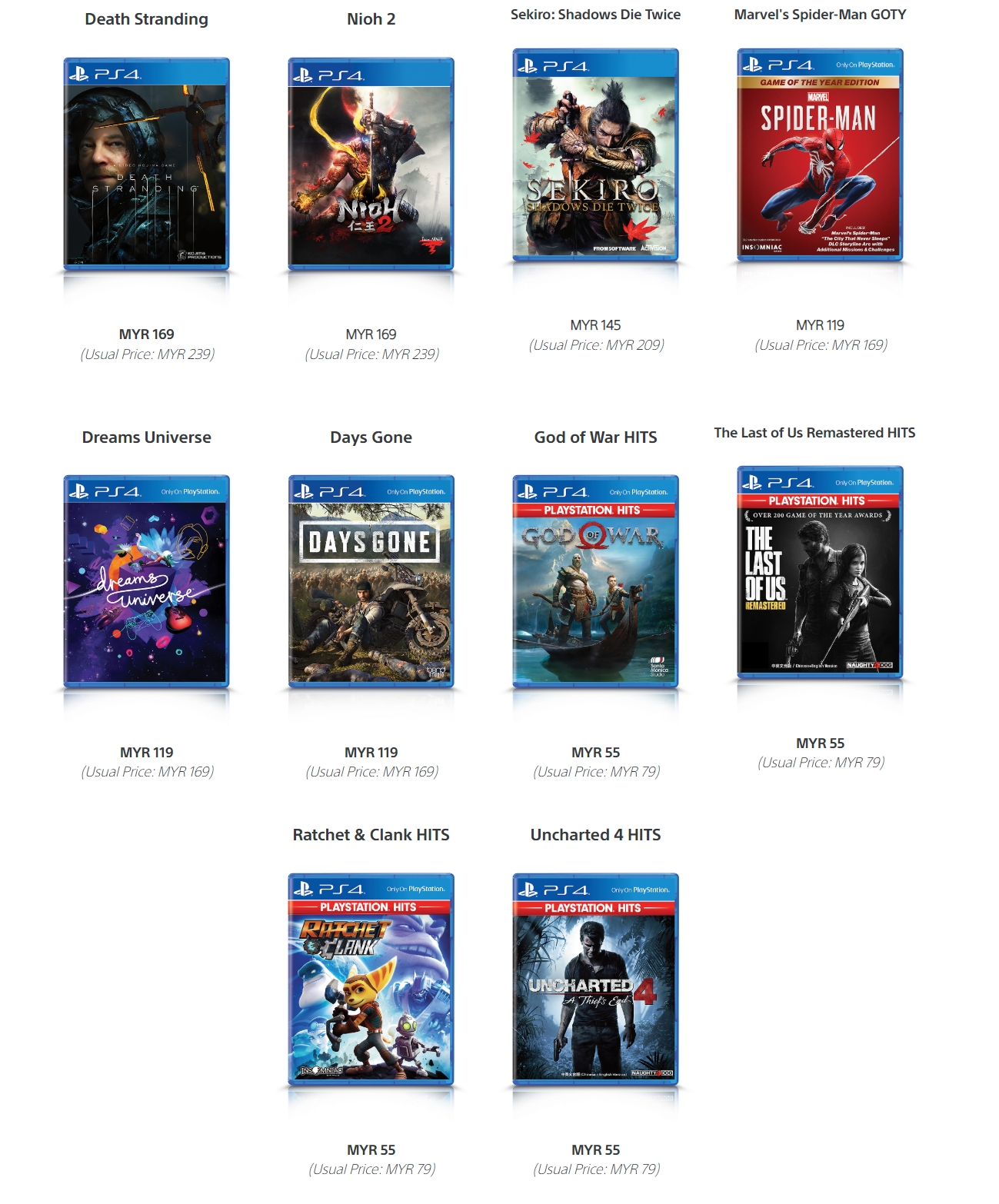The image displays a selection of PlayStation 4 game thumbnails along with their prices, organized in three horizontal rows. The first row consists of four games: "Death Stranding," "Nioh 2," "Sekiro: Shadows Die Twice," and "Marvel's Spider-Man: Game of the Year Edition." In the second row, there are also four games: "Dreams Universe," "Days Gone," "God of War: Hits," and "The Last of Us Remastered: Hits." The third row features two games: "Ratchet & Clank: Hits" and "Uncharted 4: Hits." Prices are as follows: "Death Stranding" is listed at MYR 169, "Nioh 2" at MYR 169, "Sekiro: Shadows Die Twice" at MYR 145, and "Marvel's Spider-Man: Game of the Year Edition" at MYR 119. The remaining games do not display visible prices in this image.